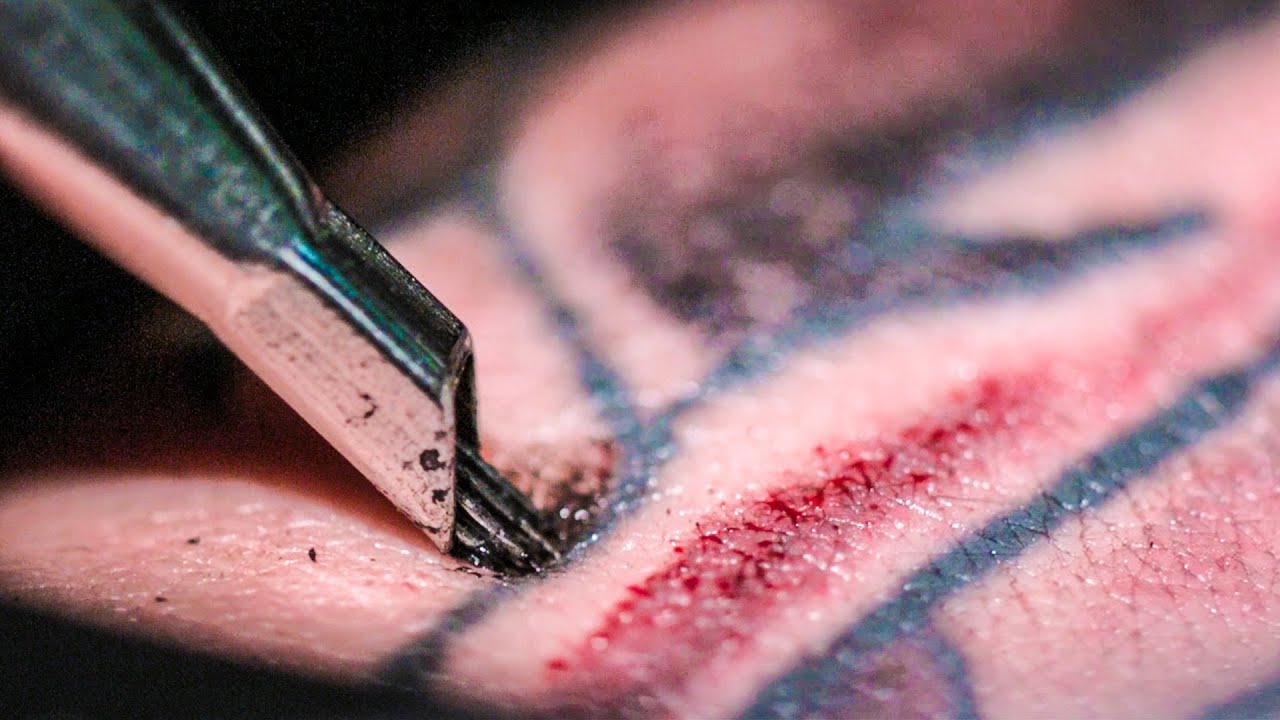The image is an extremely close-up view of a tattoo being applied to a human arm. The skin, featuring a pinkish tone, is depicted in great detail, showing a mix of blue and red ink lines, and some areas exhibit signs of redness and slight bleeding. A tattoo needle, the central focus, is seen pressing into the skin, actively injecting black ink into the intricate lines of the design. The surrounding areas of the skin and parts of the image are slightly blurred due to the extreme zoom, but the meticulous process of tattooing stands out vividly against the dark background.